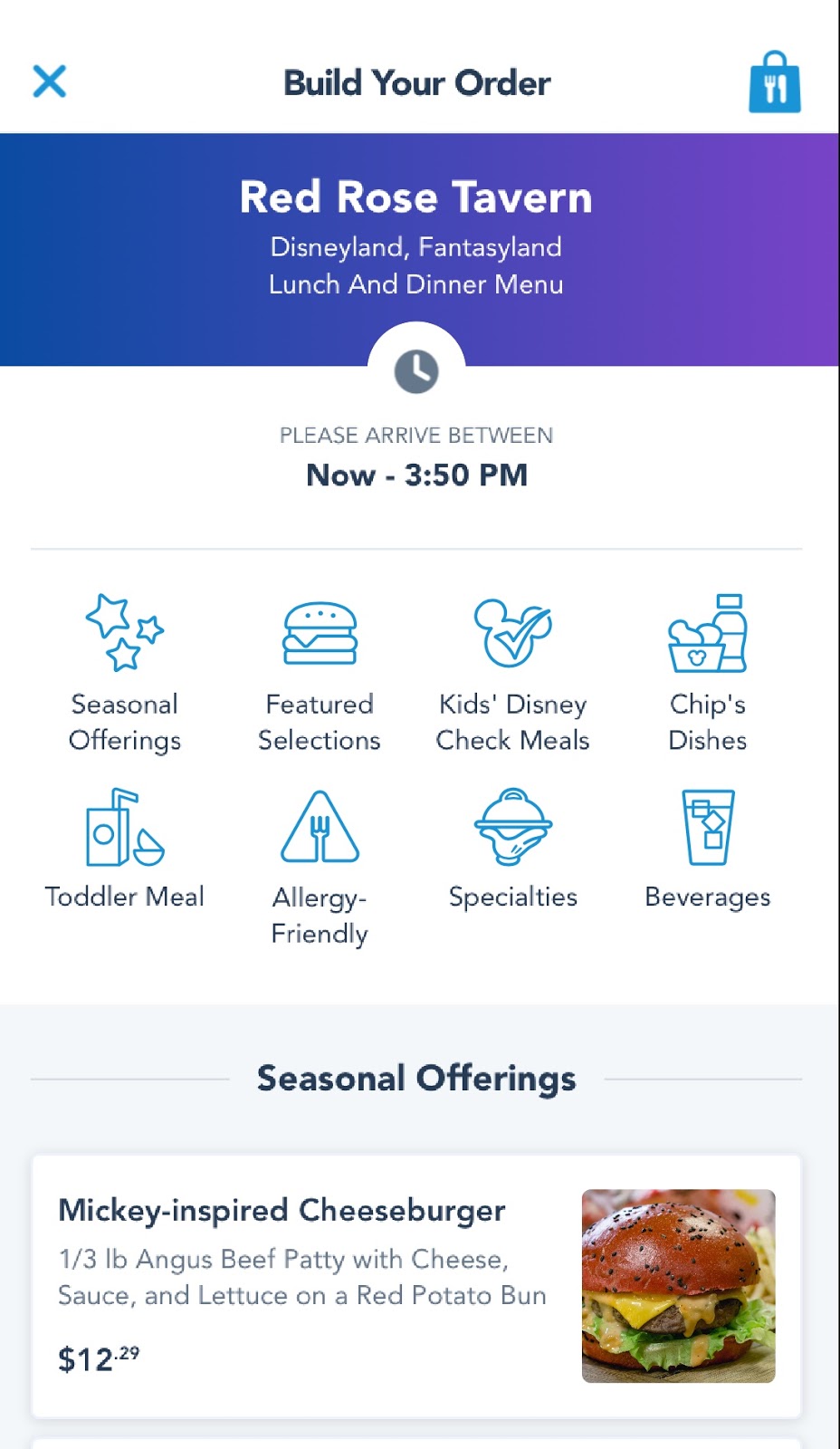The image showcases a web page for the Red Rose Tavern. The title "Red Rose Tavern" is prominently displayed in bold white font on a purplish-blue rectangular background. Directly below, in a smaller, lighter font, it reads "Disneyland, Fantasyland," followed by "Lunch and Dinner Menu." 

To the side, there is a small clock icon showing the time at 4 o'clock. Accompanying this, the text instructs, "Please arrive between now – 3:50 p.m."

Further down, the web page features icons for various menu categories such as Seasonal Offerings, Featured Selections, Kids' Disney Check Meals, Chips, Dishes, Toddler Meal, Allergy-Friendly Specialties, and Beverages.

Beneath these icons is a bold black rectangular header labeled "Seasonal Offerings." Directly underneath, within a white rectangle, the text "Mickey-inspired cheeseburger" is displayed in bold font. A detailed description follows in lighter font: "One-third pound Angus beef patty with cheese, sauce, and lettuce on a red potato bun," priced at $12.29. An image of the cheeseburger accompanies the description.